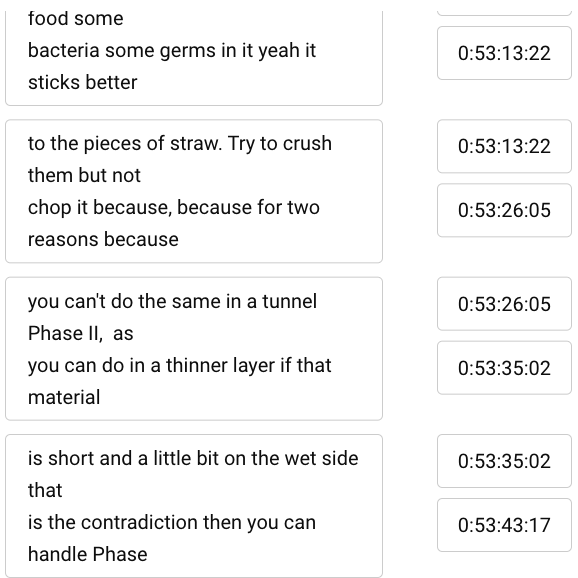The image consists of two sets of boxes arranged side by side on the screen. On the left side, there are four boxes, each containing a brief descriptive text. Correspondingly, on the right side, there are boxes featuring sequences of numerical stamps, which seem to be associated with the text on the left. Each pair is surrounded by a thin gray box, making everything clear and easy to read.

1. The first text box reads: "Food with some bacteria and germs—sticks better." Adjacent to it is a numerical box displaying: "0..5, 3..1, 3..2."

2. The second text box states: "To pieces of straw—try to crush them but not chop, for two reasons." The corresponding numerical box contains: "53 13 22" and "53 26 05."

3. The third text box indicates: "You can't do the same in a tunnel phase 2 as you can in a thinner layer." The adjoining numerical box reads: "53 26 05" and "53 35 02."

4. The final text box says: "Short and a little bit on the wet side is the contradiction that you can't handle phase." The linked numerical box shows: "53 35 02" and "53 43 17."

There are no other images present in the screenshot. The information layout is precise and well-organized, with clear and legible text and number stamps in thin gray boxes.